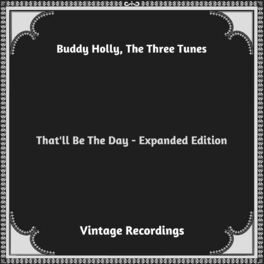The image is a cover of a vintage music record featuring Buddy Holly and The Three Tunes. The design is square with a narrow border of black and gray stripes. Inside this border, a solid black rounded shape serves as the background for three lines of white text. At the top, it reads "Buddy Holly, The Three Tunes." The center line states "That'll Be the Day - Expanded Edition," and the bottom line reads "Vintage Recordings." This detailed and stylish layout creates an attractive visual that emphasizes the timeless nature of the recordings.